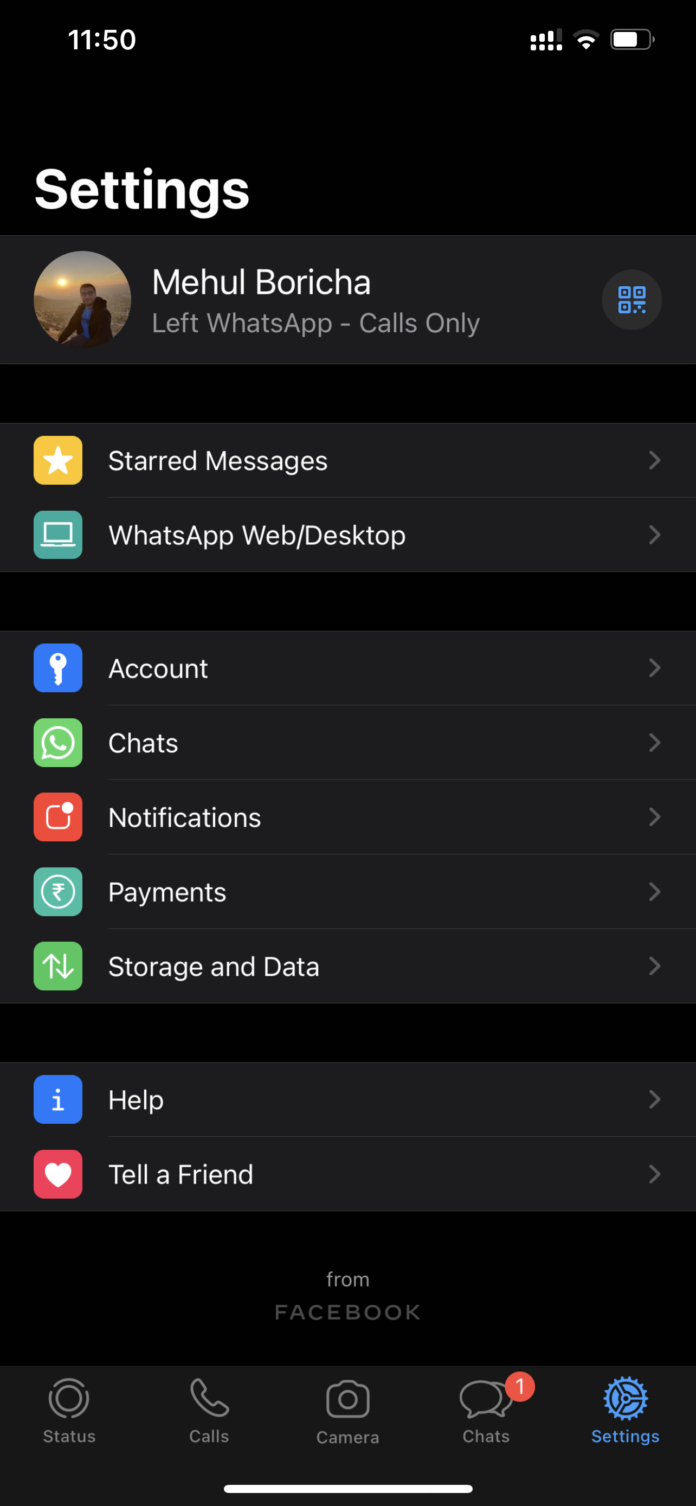The image is a screenshot taken from a cellphone, showing the settings interface of the WhatsApp application. The background of the screen is entirely black, providing a stark contrast to the white text and icons displayed.

At the very top of the image, the time "11:50" is prominently featured in white text. To the right of the time, signal bars indicating cellular reception and a Wi-Fi icon can be seen, followed by a battery icon that is approximately two-thirds charged, with the battery partially filled in white and the remaining section blank.

Beneath this top information bar is a section labeled "Settings" in white text. Directly underneath this label is a profile picture of a man illuminated by the light of a setting sun, with the username Mahool Boricha displayed adjacent to the image. Below the username, it is noted that this individual prefers "WhatsApp - calls only."

Continuing downward, there are several icons and corresponding captions lined up on the left side of the screen. The first section includes two items:
1. A star icon beside the label "Starred Messages."
2. A computer within a box icon beside the label "WhatsApp Web - Desktop."

This section is separated by a black line, followed by a group of five more items:
1. "Account"
2. "Chats"
3. "Notifications"
4. "Payments"
5. "Storage and Data"

Another black line segregates this group from the final set of options, which includes "Help" and "Tell a Friend" placed at the bottom.

Overall, the image captures a detailed view of various setting options available within the WhatsApp application, highlighting the user's profile and preferred app usage.